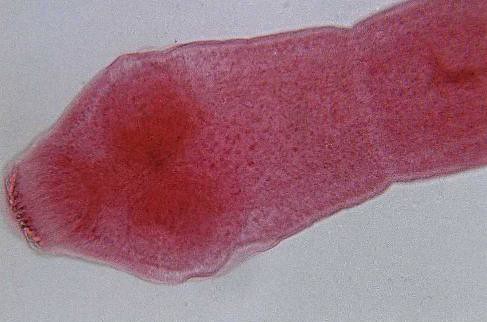The image depicts a magnified microscopic view of what appears to be an amoeba or a similar small, microscopic creature. It features a long, snake-like shape with an asymmetrical and random pattern. The creature exhibits a predominant red color with varying shades, including light red to deep red and touches of pale pink near its extremities. The left side of the form, which could be interpreted as the head, shows darker red shading, somewhat resembling eyes and a mouth. The entire organism is set against an off-white or light gray background. The image is slightly blurry, emphasizing the magnified, extreme close-up nature of the shot.